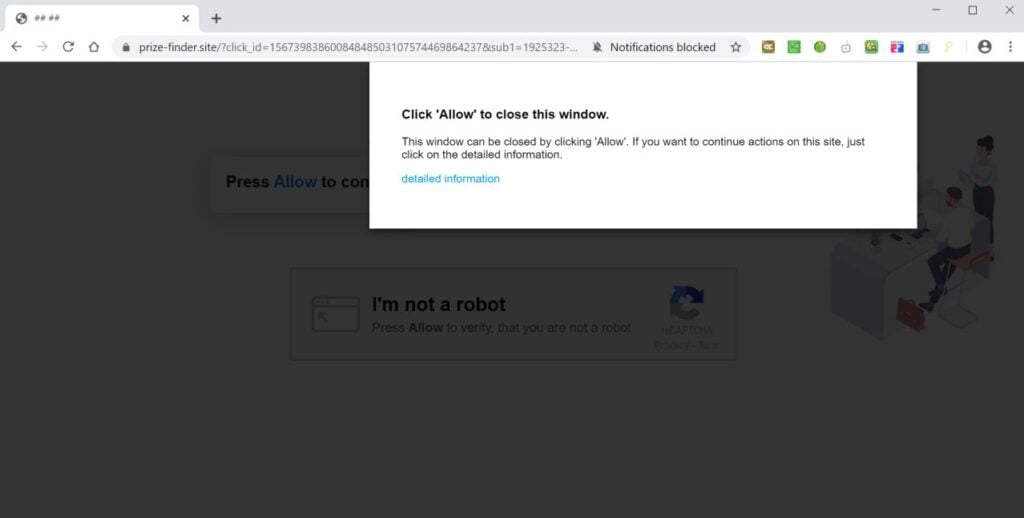The screenshot is predominantly blacked out, obscuring much of the background content. A noticeable white pop-up occupies the central position, partially overlaying the grayed-out main background, which has minimal visible text. Within the white pop-up, bold black text reads: "Click Allow to close this window." Below this, additional instructions state: "This window can be closed by clicking Allow. If you want to continue actions on this site, just click on the detailed information." A blue hyperlink text labeled "detailed information" is found at the bottom of the pop-up.

Embedded within the background, partially visible text includes a CAPTCHA challenge stating, "I'm not a robot," with a directive to "press allow to do something" underneath. To the right of the CAPTCHA, there appears to be an image featuring a man seated at a desk with a woman standing beside him.

At the top of the screenshot, the browser's taskbar is evident, displaying common navigation elements like arrows, a home icon, and a search bar. A notification indicating "Notifications blocked" can be seen, along with various colored and shaped icons whose meanings are not specified. Above the taskbar, the browser tab bar is visible, showing an open tab with an Earth icon, an "X," and a "+" sign. The browser window's control bar above the tab includes standard minimize, maximize, and close buttons, represented by a gray bar with the respective symbols: minus, square, and X.